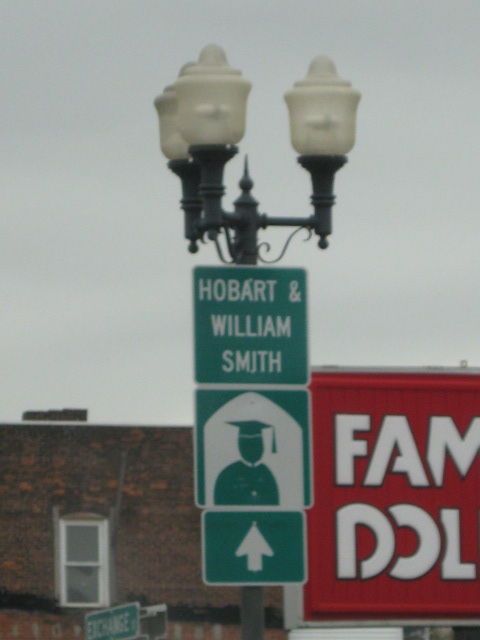This photograph captures a vibrant street scene in front of a business establishment under a cloudy gray sky. Dominating the frame is a large, partially visible red storefront sign with white lettering reading "FAM" and "DOL," which appears to be for a Family Dollar store. Adjacent to this, a green street sign with a white border features an upward-pointing arrow leading to a white archway depicted with an image of a graduate. Above this, the sign is labeled "Hobart and William Smith" in white print. The scene is anchored by a brown and orange brick building in the background, adorned with a white-trimmed window. Three distinct lights, mounted on black brackets, illuminate the area with their white glass canisters enclosing the bulbs. The gray post supporting the signs adds a touch of utilitarian structure to the rich visual narrative.